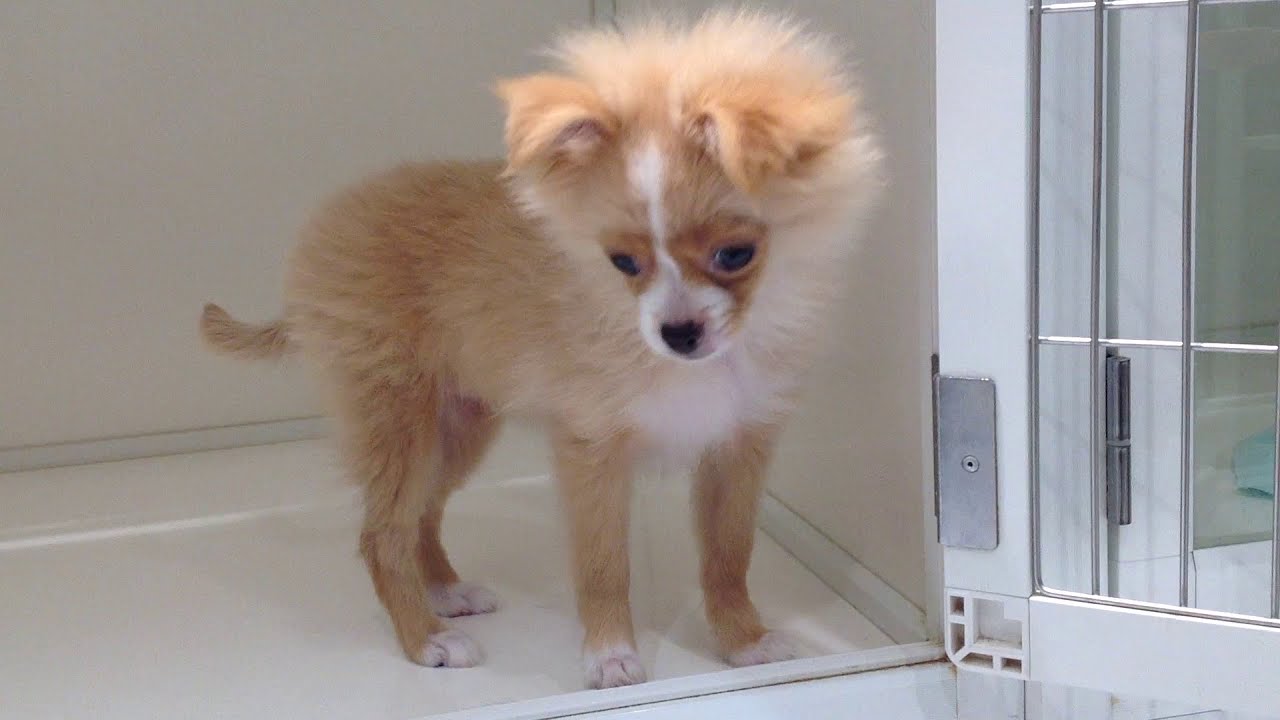The image is a detailed digital photograph taken inside a pet shop, focusing on a small dog, likely a mix between a Pomeranian and a Chihuahua, standing inside an open white cage. The dog has a fluffy light brown coat with prominent fluff around its head, face, and chest, accentuated by white patches on its chest and paws. Its head, featuring a small triangular face, black nose, and striking round black eyes, is slightly tilted downward as it gazes intently at something outside the cage. The dog's eyes are bordered by a darker patch that highlights its expressive features, and a line of white fur runs from between its eyes to its forehead. The open door of the cage has a white frame with thin silver wires. Adjacent to the dog's cage is another cage with a teal blanket on the floor, providing depth and context to the setting. The backdrop and floor inside the cages are white, enhancing the visual focus on the dog's detailed coat and expressive eyes. The overall color scheme of the photograph includes shades of brown, white, gray, silver, and teal.